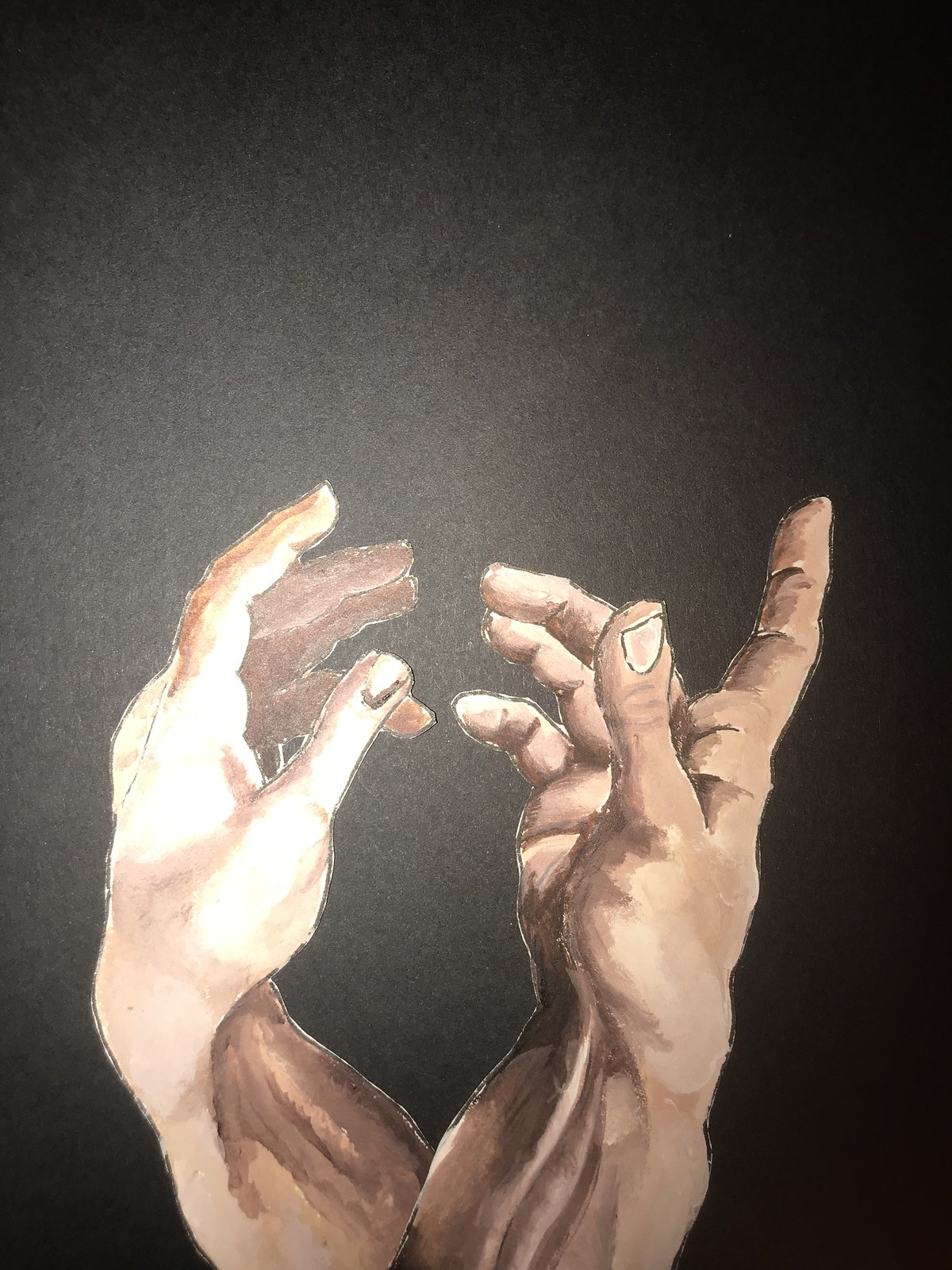This slightly vertical watercolor painting vividly captures two hands reaching toward each other, positioned diagonally and bending at the wrists. The left hand, with its longer, narrower fingers and smaller fingernails, appears slightly feminine. In contrast, the right hand, displaying shorter and broader thumbs and larger fingernails, exudes a masculine quality. Both hands are depicted in a harmonious palette of browns, light tans, and ochre tones. The pointer fingers are somewhat extended while the remaining fingers are gently bent, and the thumbs are turned upward.

Set against a stark black background, the composition draws the viewer's focus to the hands, accentuated by a subtle highlight in the center that may either reflect the light source or the artist's intention to create a halo effect. The image is cropped mid-forearm, with the hands extending from the lower center towards the upper center, creating a dynamic and evocative visual connection.